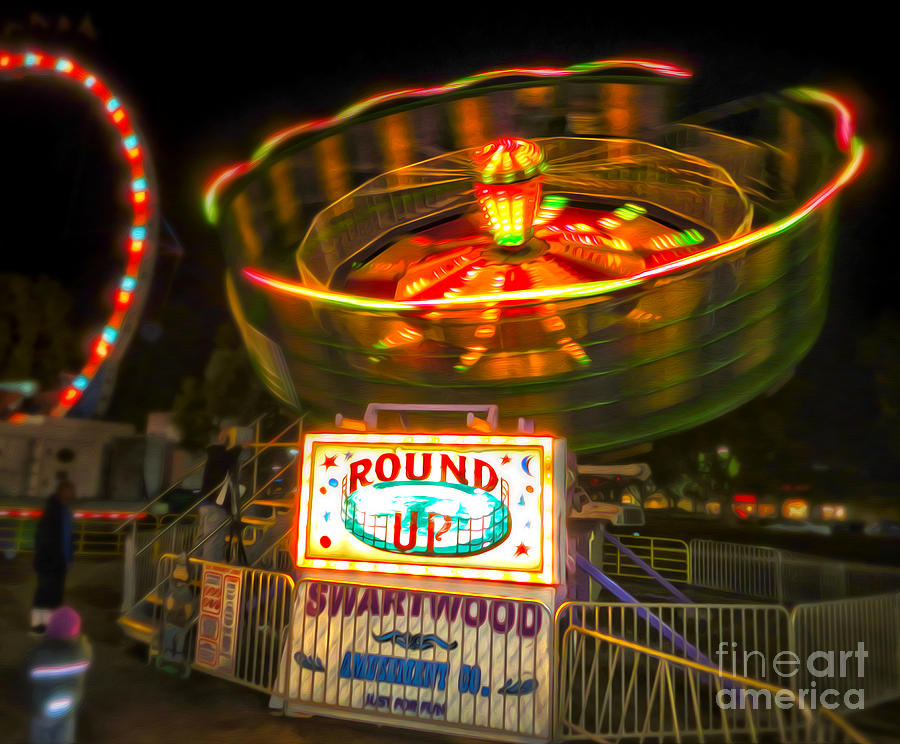The square image captures the vibrant energy of an amusement park at night. Dominating the scene is a spinning ride called "Round Up," evidenced by a prominently lit sign in red letters situated just behind a metal gate. The ride itself is a circular contraption with a spinning center, likely one that uses centrifugal force to press riders against the walls. The sign also features the word "Swartwood" beneath "Round Up," accompanied by some blue text that is too blurry to discern clearly. 

The background reveals a blurry but colorful ferris wheel on the upper left, illuminated in red, orange, and blue hues. A figure clad in dark clothing stands on the left side of the image, another person wearing a glowing coat and pink hat appears in the lower left. The picture bears the watermark "Fine Art America" in light gray letters in the lower right corner. The overall blur and lighting suggest the image captures the dynamic motion and excitement of the amusement park at night.